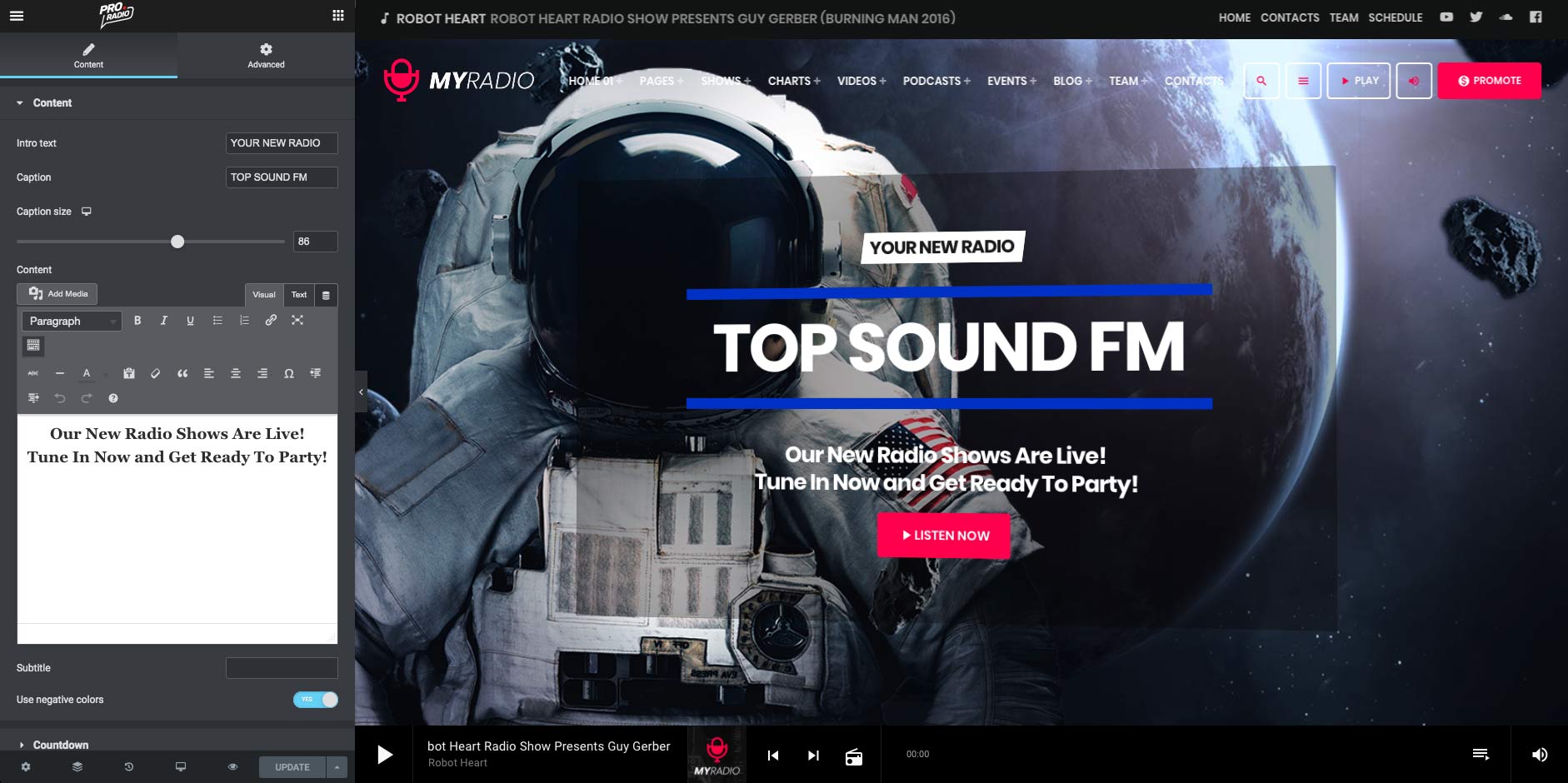The screenshot captures a visually engaging media application designed for music and entertainment consumption. Centered prominently on the homepage is a striking image of an astronaut, depicted from the waist up. The astronaut's attire features a visible American flag patch on the sleeve, a dark visor on the helmet obscuring any facial features, and a backpack. The backdrop consists of a slightly faded celestial scene, possibly of Earth, complemented by stars and asteroids, enhancing the space theme.

Superimposed over the astronaut image is a vibrant window that invites users to engage with "Top Sound FM." The text announces, "Your new radio shows are live, tune in now and get ready to party," accompanied by a clickable button labeled "Listen Now." This overlay is the focal point of the application, emphasizing its radio streaming capabilities.

Running horizontally across the top is a navigation menu that prominently displays "My Radio," the probable name of the application. The menu includes various options such as Charts, Videos, Podcasts, Events, Blog, Team, and Contact. Additionally, there are essential controls like play/stop, search, and volume buttons.

On the left-hand side of the homepage, there is a search box designed for users to find specific content and customize their media preferences. This snapshot of the application highlights its primary focus on music while also offering a diverse array of media including videos, podcasts, and live streams. The astronaut image serves as a distinctive and memorable background, creating a captivating entrance to the site.